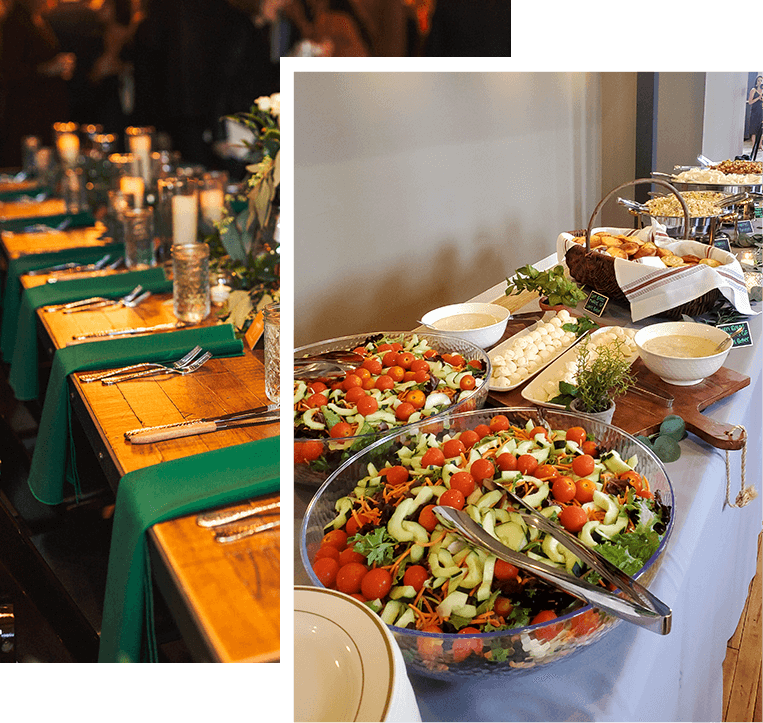The image is composed of two photos placed side by side, showcasing an elegant dinner setting and an assortment of delectable foods, evoking a sense of luxury and meticulous attention to detail.

**Left Photo:**
A sumptuous wooden table is adorned with an array of crystal glasses and softly glowing candles. Some of the crystal glasses are artistically filled with flowers, adding a touch of natural beauty to the setting. Each place setting is meticulously arranged with shiny silverware and green napkins that gracefully hang off the edge of the table, enhancing the table's sophisticated appearance.

**Right Photo:**
On a table draped with a pristine white tablecloth, an enticing variety of foods are artfully presented. Clear bowls contain vibrant salads, and white bowls hold what appears to be a rich soup or sauce. A basket brimming with fresh bread invites guests to indulge. In the far background, several pizzas add a delightful rustic touch. Centrally positioned on the table are white round objects on white platters, further accentuating the harmonious blend of colors and textures in the display. 

The juxtaposition of the elegant table setting and the lavish spread of culinary delights creates an inviting atmosphere, perfect for a memorable dining experience.